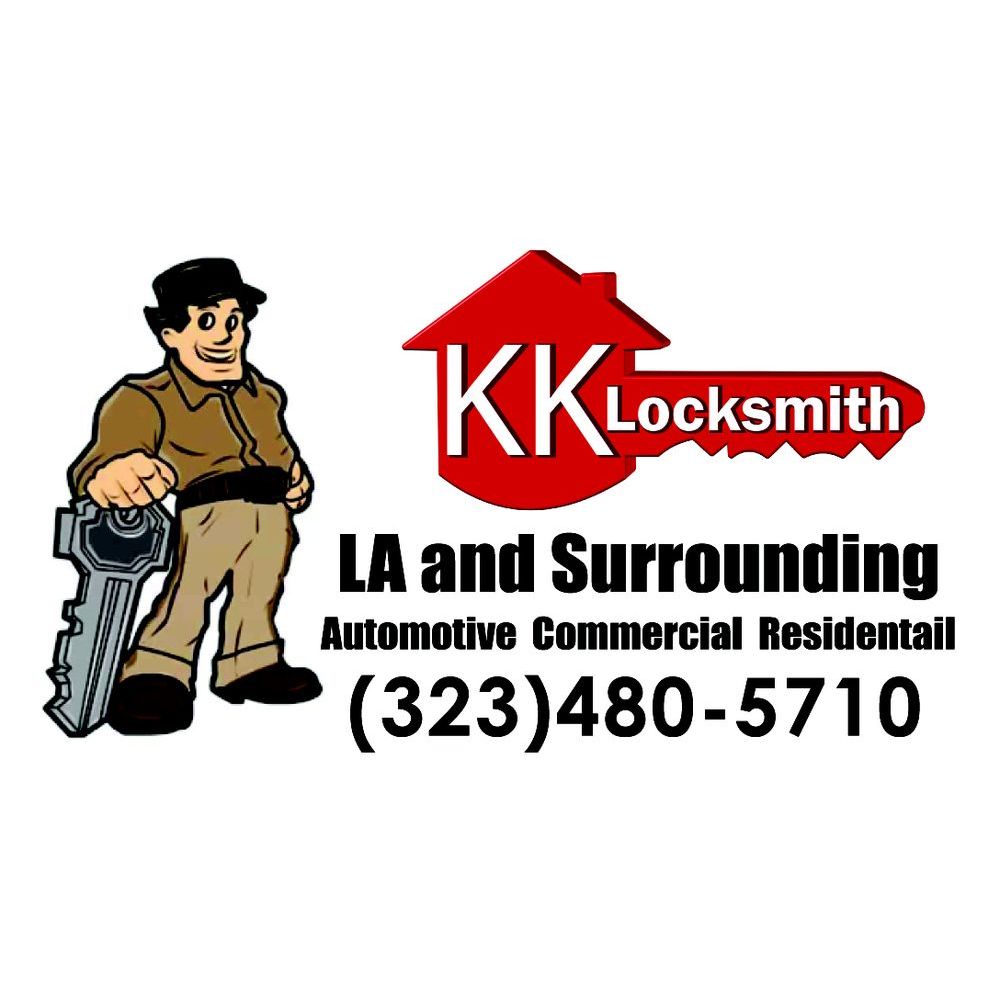The image is an advertisement for "KK Locksmith," prominently featuring a logo and a cartoon character. The character, a powerful-looking locksmith, is illustrated on the left side, wearing a brown uniform, beige pants, brown shoes, and a brown hat, with black hair. He is smiling and appears to be resting a large silver key on the ground like a cane.

To the right of the character is a large red key, where the handle is shaped like a house. Superimposed on this red key, in white text, is the name "KK Locksmith." Underneath, in black text, it reads, "LA and surrounding, automotive, commercial, residential," followed by the phone number "323-480-5710." The entire design effectively combines essential details to advertise comprehensive locksmith services.